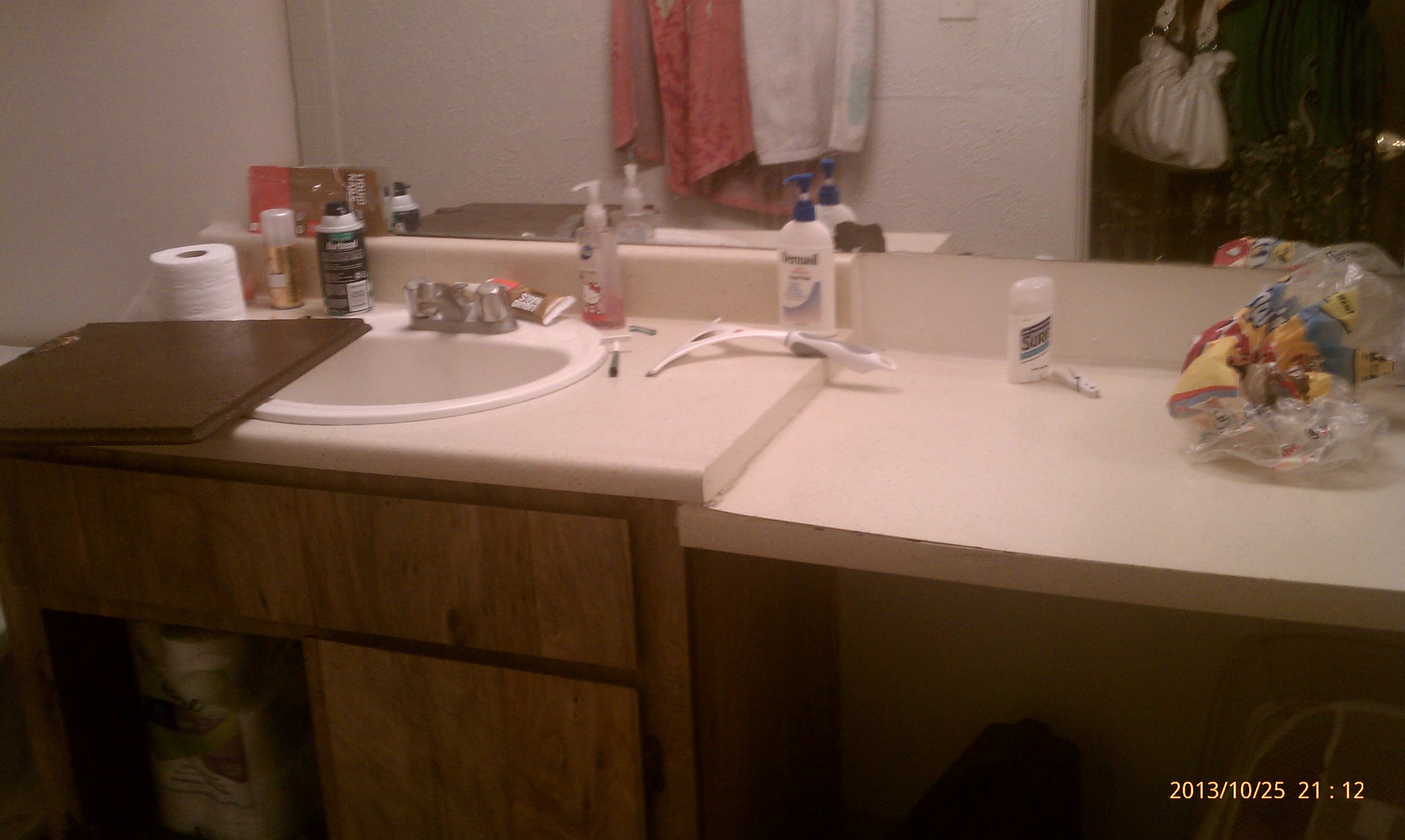This color photograph, dated October 25, 2013, at 21:12, captures a dual-level bathroom sink area, offering a blend of functionality and style. The upper countertop houses a white sink with a sleek silver faucet, embedded in an off-white or light taupe laminate surface with smoothly rounded edges and an integrated splashback. Below this sink level, a secondary countertop sits lower, designed possibly for use as a dressing table, providing easy access for sitting.

The area features brown wooden cabinetry under the sink section, while the right side, corresponding with the lower countertop, is open to allow for a chair, creating a convenient makeup area. A full-length mirror spans the wall behind the sink and dressing table, reflecting the neat arrangement of towels hanging nearby. Various soaps and personal care products are neatly placed on the countertops, completing this efficient and aesthetically pleasing bathroom setup.